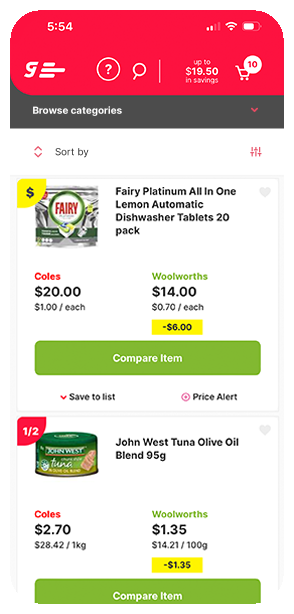The screenshot captures the user interface of a shopping app at 5:54 PM, as indicated by the time displayed at the top. The red header area features various icons, including a "G" with three white lines to its right, a question mark in a circle, a magnifying glass for search functionality, and a cart icon with the number 10 beside it, indicating items in the shopping cart. Below the header, a banner promotes "up to 1950" in savings.

In the black area beneath that, there's an option to "Browse Categories," flanked on the right by a "Sort By" button with three horizontal lines for menu access.
 
The app displays a list of items, the first being "Fairy Platinum All-in-One Lemon Automatic Dishwasher Tablets, 20 pack." An image of the product packaging, featuring the brand name "Fairy," is included. The product pricing is compared between two stores: Kohl's offers it for $20 or $1 per tablet, while Woolworths lists it for $14 or $0.70 per tablet. A yellow icon indicates a $6 discount, and a green button allows users to "Compare Item." Below this are options to "Save to List" and set a "Price Alert."

The next item is "John West Tuna Olive Oil Blend, 95g," accompanied by a green product image. Highlighted in red is a "Half Off" deal. Price comparisons show Kohl's at $2.70 and Woolworths at $1.35, with a yellow icon indicating a $1.35 discount. A green "Compare Item" button is also present.

Overall, the screenshot provides a detailed and organized interface for comparing product prices and managing shopping needs.